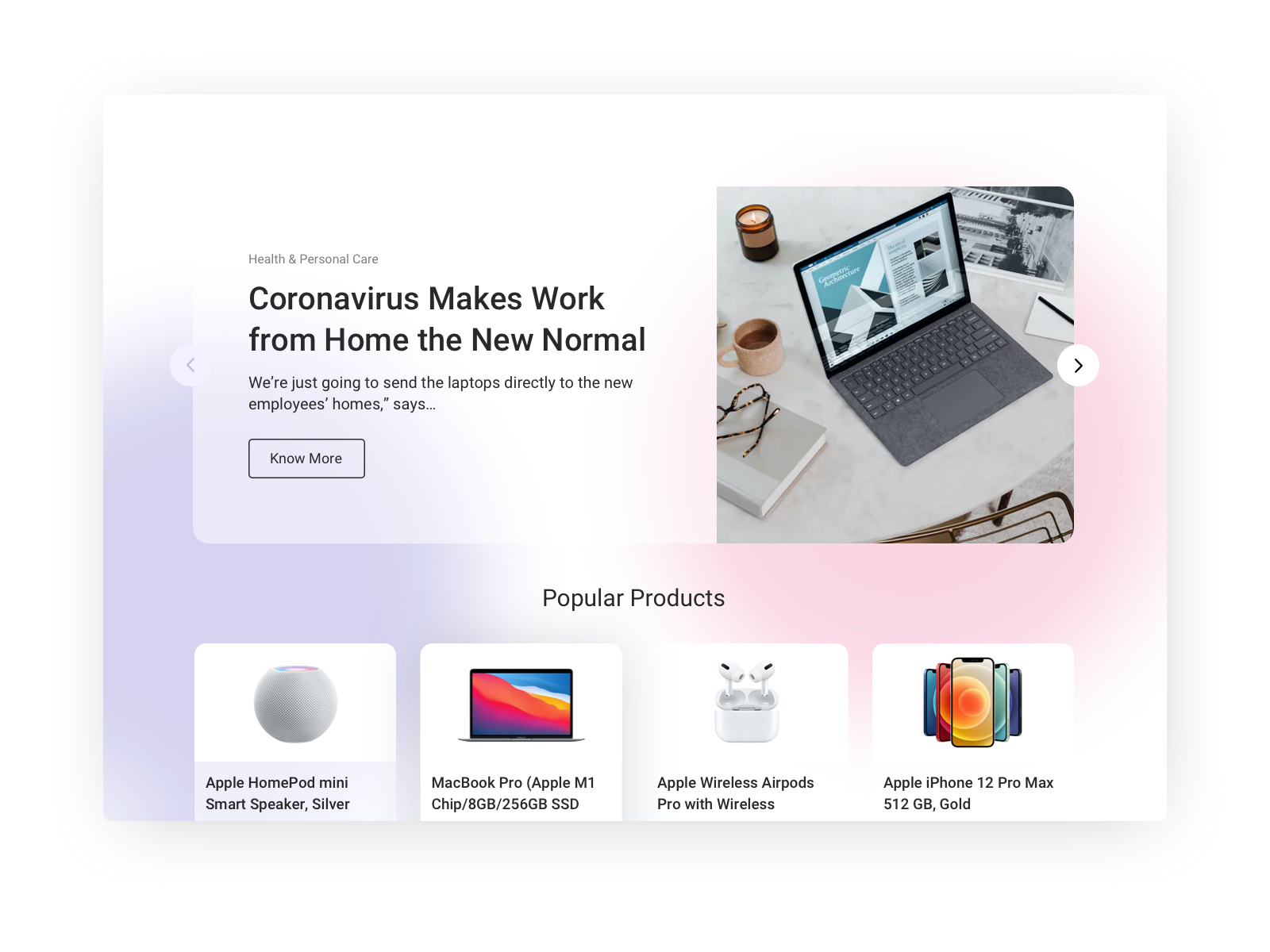**Detailed Caption:**

A screenshot of an advertisement captures the shift toward remote work due to the coronavirus pandemic. The central text on a white background, in bold black font, reads "Coronavirus makes work from home the new normal." Above this, positioned to the left in small, light gray font, the category is marked as "Health and Personal Care." Just below the main message, a smaller black font displays a quote: "We're just going to send the laptops directly to the new employees’ homes…" followed by an ellipsis.

The bottom half of the image features a cozy work-from-home setup. On the right, an open laptop sits on a tabletop, displaying a web page. Beside it, there's a lit candle and a steaming cup of coffee, lending a comforting ambiance to the workspace. A book with eyeglasses placed on top adds a touch of personal touch to the scene. Nearby, a few pictures, a piece of paper, and a pen are neatly arranged, further emphasizing a well-organized work area. Although the chair isn't visible, its presence is implied in front of the table.

In the lower right-hand corner, small directional arrows point left and right, suggesting navigation options. Below the workspace depiction, the text "Popular Products" introduces a section showcasing four popular items, each presented in individual white background boxes. These products include the Apple HomePod mini smart speaker (silver), a MacBook Pro with Apple M1 chip (8GB RAM, 256GB SSD), Apple AirPods Pro with wireless charging, and an Apple iPhone 12 Pro Max (128GB, gold).

The entire background of the screenshot is a soft, blended gradient of purple, white, and pink hues, creating a visually pleasing ombre effect that ties the advertisement together.